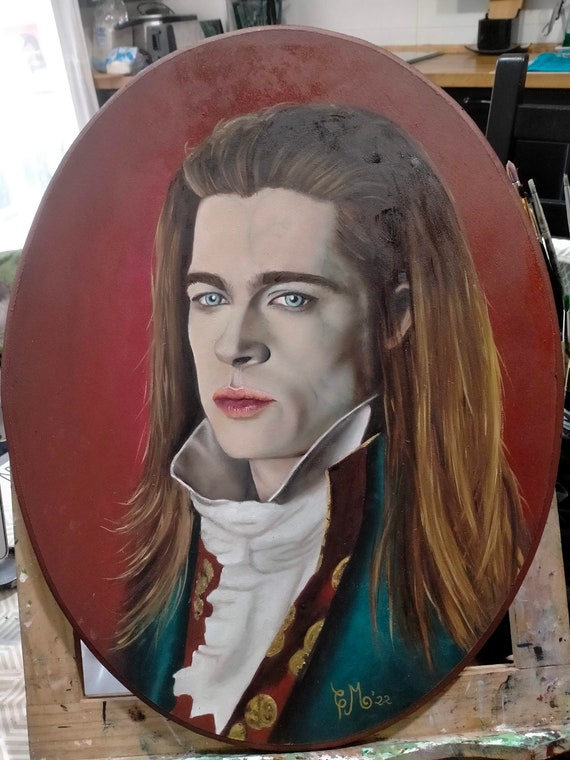This is an intricate painting expertly capturing Brad Pitt's character from "Interview with the Vampire." The portrait, framed within an oval-shaped red canvas, prominently features a man with long, light brown hair, pale skin, and expressive icy light blue eyes. His lips are strikingly red, and he wears a classic white collared shirt beneath a dark green suit jacket adorned with red lapels and gold buttons. The background of the painting is a rich, deep maroon.

The setting of the image suggests an artist's studio or a home, with the painting positioned on a wooden stand. In the background, various kitchen counters are visible, displaying small appliances, paintbrushes on the right, and other devices, creating a lived-in, creative atmosphere. Below the ornate red frame of the painting, there is an additional plain wooden frame with nothing in it. A subtle autograph, potentially containing the letters 'C,' 'G,' and 'M,' followed by '22', is located at the bottom right of the painting, further emphasizing its unique character and artistic value.